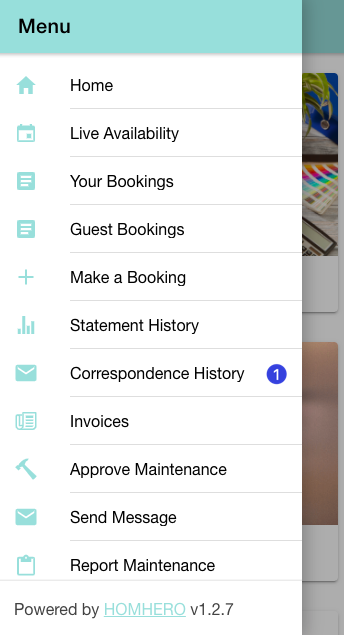The image showcases a menu from an application. The top section of the pop-up menu window is light green, featuring the word "Menu" in black, capitalized font. Below this light green bar, the menu is organized into a vertical list with each item accompanied by an icon on the left. 

1. **Home** - Represented by a home icon.
2. **Live Availability** - No additional icon mentioned.
3. **Your Bookings** - Indicated by a page icon.
4. **Guest Bookings** - Also marked with a page icon.
5. **Make a Booking** - Identified by a plus sign icon.
6. **Statement History** - Illustrated with a bar graph icon.
7. **Correspondence History** - Denoted by an email icon, which has a blue circle containing the number 1 in white font.

The menu layout is intuitive and provides quick access to various functions of the app.